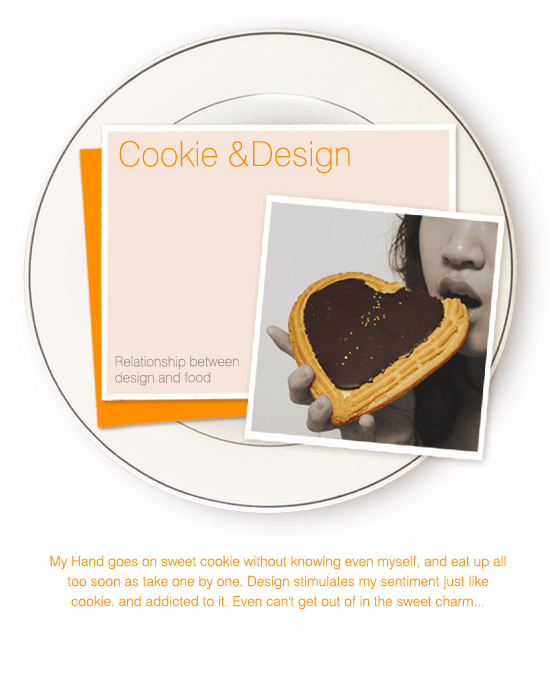The image features a circular plate outlined in black with an irregular circumference. Overlaid on this plate are three square cards arranged in a stacked manner. The bottom card, partially visible, is orange with only its left and bottom edges showing. On top of this is a pink card with a white outline, displaying the text "cookie and design" in orange letters on the top left, and in smaller black letters at the bottom left, "relationship between design and food." The right portion of this pink card is obscured by the topmost card. The uppermost card is a photograph outlined in white, depicting a woman with long black hair. She is cut off above her nose and to the right of her mouth, and she is holding a heart-shaped pastry or cookie with chocolate frosting up to her mouth. Beneath this composition, there are three lines of orange text that read: "my hand goes on sweet cookie without knowing even myself and eat up all too soon as take one by one. Design stimulates my sentiment just like cookie and addicted to it. Even can't get out of in the sweet charm..."